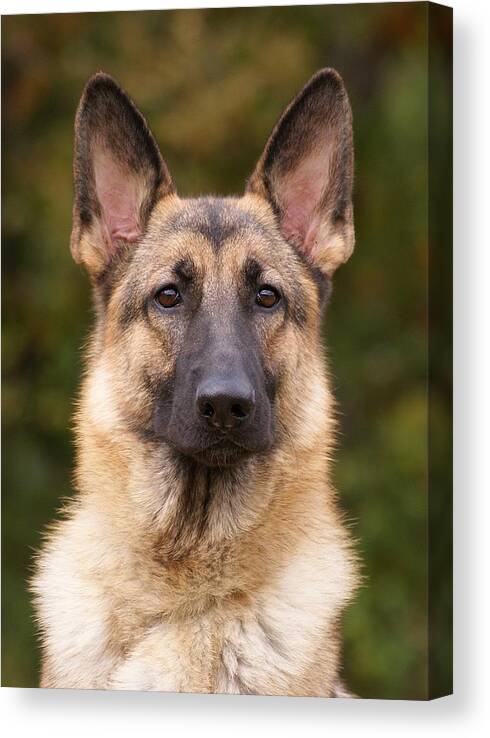This detailed photograph captures a majestic German Shepherd from the shoulders up, set against a background of blurred green vegetation. The dog's alert and expressive face is perfectly in focus, highlighting its striking features. It is seated, facing slightly toward the right of the frame, with ears perked up and pointed skyward, revealing pinkish interiors. The German Shepherd showcases a beautiful coat of light tan or cream, accentuated by patches of black on its snout, around the eyes, forehead, and the tips of its ears. Its eyes are a deep, soulful brown. The jowls and neck area possess tufts of white fur that extend down to the visible part of its body. The image has a three-dimensional quality, seemingly making the dog pop out, with a subtle shadow effect emphasizing its contours. The background, though out of focus, hints at a natural environment with hues of green, yellow, and hints of orange. This creates a beautiful contrast to the sharp clarity of the dog's features, making it the captivating focal point of the image.